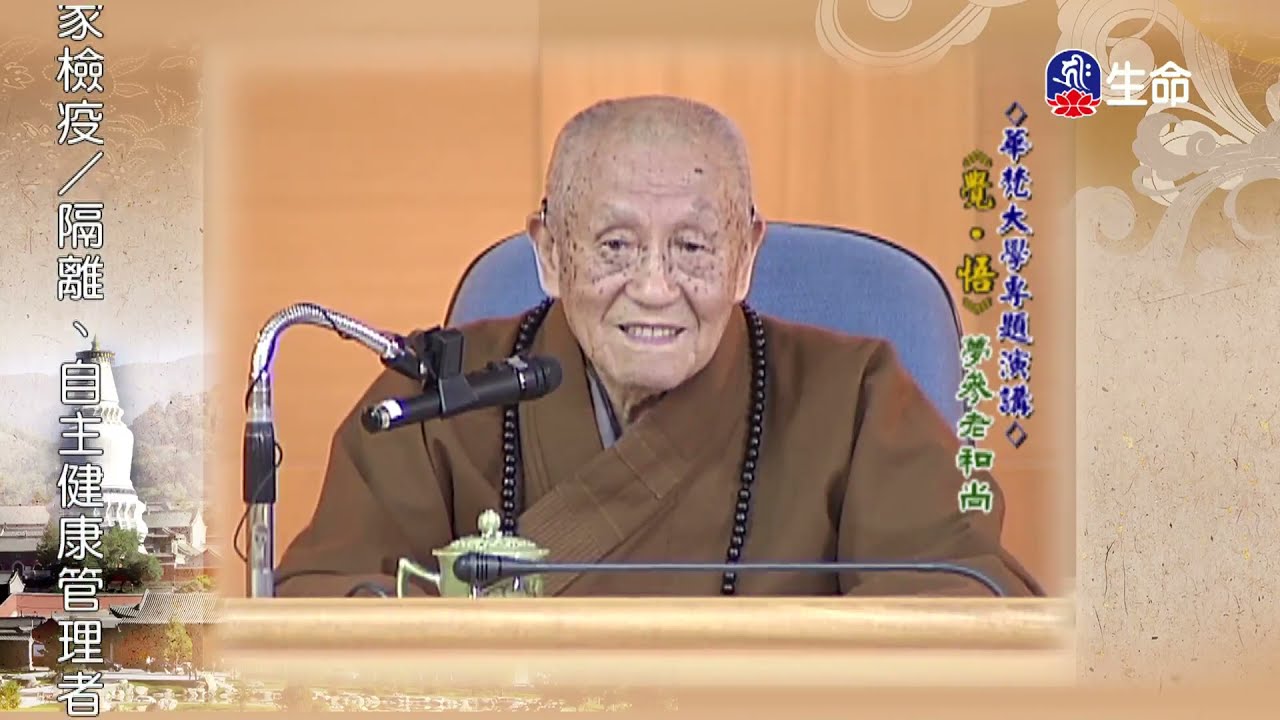In the image, there is an elderly, bald monk with pale skin and numerous freckles on his face, seated solemnly on a blue chair. The monk, who appears to be in his late 70s or 80s, wears a brown robe that crosses over his chest and a necklace made of black beads. Before him is a black microphone with a silver stand and a pale green cup with a green lid. The background features a soft ombre effect of peach and light browns. To the left and right of the monk are vertical strips of oriental characters; on the left, the characters are white, while on the right, they are blue, yellow, and green. The image also contains a logo in the upper right corner colored blue, white, and red. The monk's expression is a mix between a smile and a grimace, seemingly engaged in giving a speech or presentation.